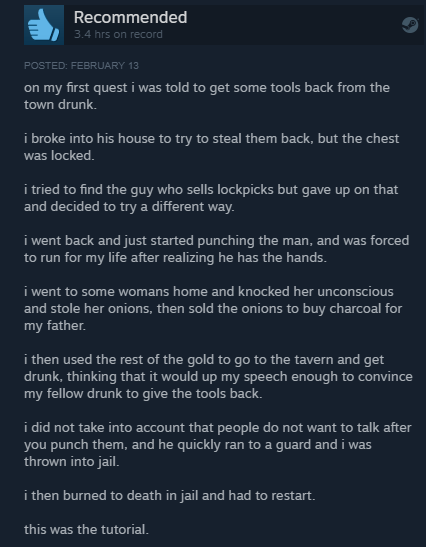This image features a screenshot from a social media post, possibly on Discord given the dark greenish-blue color scheme typical of the platform. The post, dated February 13, includes a thumbs-up icon and the label "recommended," indicating positive feedback for an activity or item with 3.4 hours recorded. All the text is presented in white and notably lacks any capitalization, even at the beginning of sentences.

The content of the post narrates a chaotic series of events within a game. The player embarks on their first quest to retrieve tools from a town drunk. Initially attempting to break into the drunk's house only to find the chest locked, the player abandons the quest for lockpicks and opts for a more direct approach. This leads to an altercation where the player punches the drunk, is overpowered, and flees.

Desperate, the player seeks refuge in a nearby woman's home, where they knock her unconscious and steal her onions. These stolen onions are then sold to purchase charcoal for the player's father. With the remaining gold, the player visits a tavern to get drunk, hoping to enhance their speech skills sufficiently to persuade the inebriated man to return the tools.

However, the player's plan backfires as previous hostile actions lead to an unwillingness for conversation from the assaulted drunk. The player ends up running to a guard, ultimately getting thrown into jail. The escapade tragically concludes with the player burning to death in jail and having to restart the game.